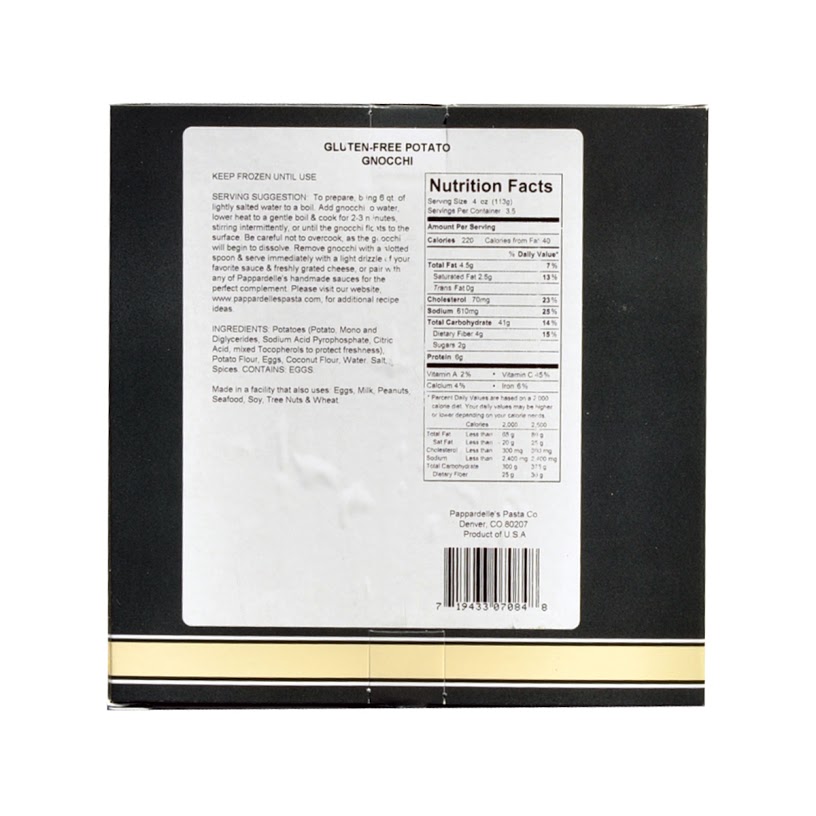This image displays the back of a package labeled "Gluten-Free Potato Gnocchi." The layout is divided into two main sections. On the left-hand side, there is a paragraph of small black text followed by the ingredients list and a concluding sentence. The right-hand side features a bold "Nutrition Facts" heading. Below this, nutritional information is organized with categories like total fat, cholesterol, sodium, etc., on the left, alongside their corresponding daily value percentages on the right. Further down, vitamin percentages are listed. The bottom of the package includes a barcode. The overall background is black, contrasted by a horizontal white strip positioned beneath the nutrition facts label.